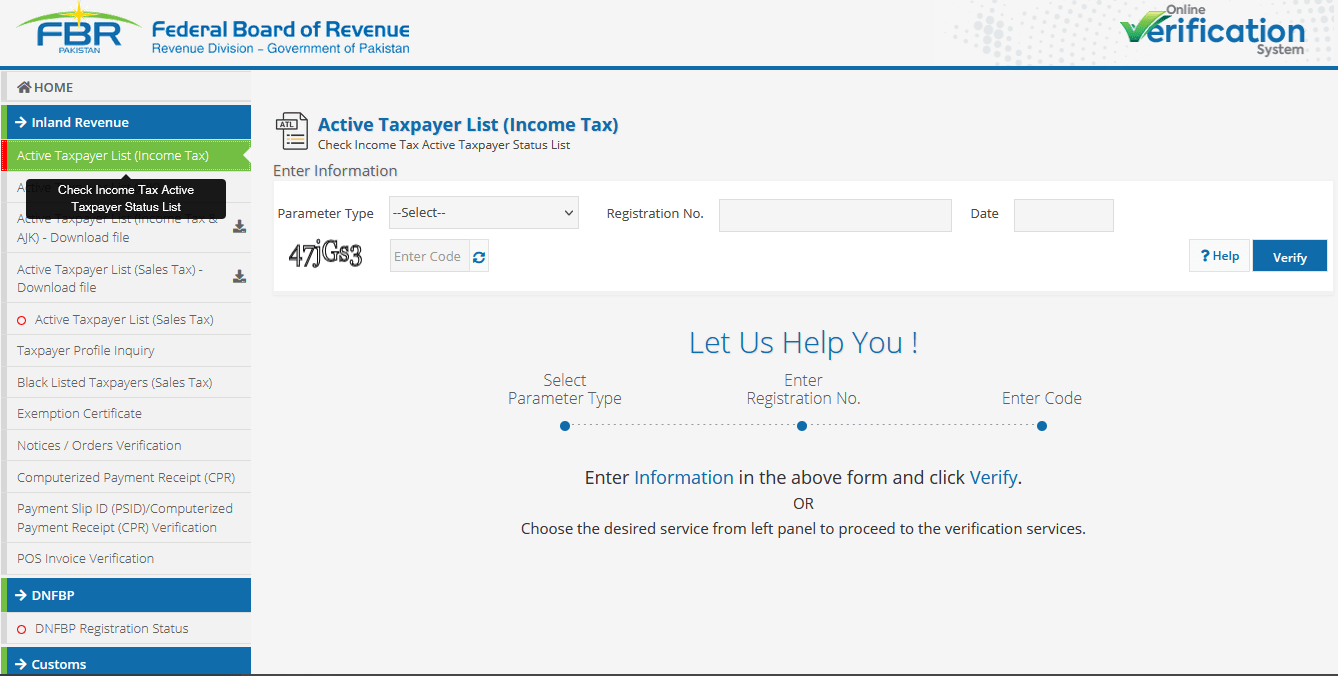The image showcases the official website of the Federal Board of Revenue (FBR), Revenue Division, Government of Pakistan, specifically featuring its online verification system. At the top, navigation options include the 'Home' button. Within the interface, various sections are organized in color-coded boxes: 

1. **Inland Revenues** in a blue box.
2. **Active Taxpayer List for Income Tax**, highlighted with a green box and a prominent red slash at its beginning. An arrow directs users to check the Income Tax Active Taxpayer Status List, emphasizing its importance.

Below these main sections, additional services are listed in blue and green boxes, such as:

- **Active Taxpayer List for Sales Tax**
- **Sales Tax Taxpayer Profile Inquiry**
- **Blacklisted Taxpayers for Sales Tax**
- **Exemption Certificate**
- **Notices**
- **Orders**
- **Verification**
- **Computerized Payment Receipt**
- **Payment Slip ID**
- **POS Invoice Verification**

Furthermore, two focused sections labeled **DNFBP** and **Customs** are also present in blue boxes. 

For user convenience, instructions are provided to check the Income Tax Active Taxpayer Status List. Users need to select the parameter type, enter the registration number, provide the date, and input a security code. An additional aid comment reads, "Let us help you. Select parameter type, enter registration number, enter code."

Users have the choice to either confirm their information through this form or select a desired service from the left panel to proceed to their specific verification requirement.